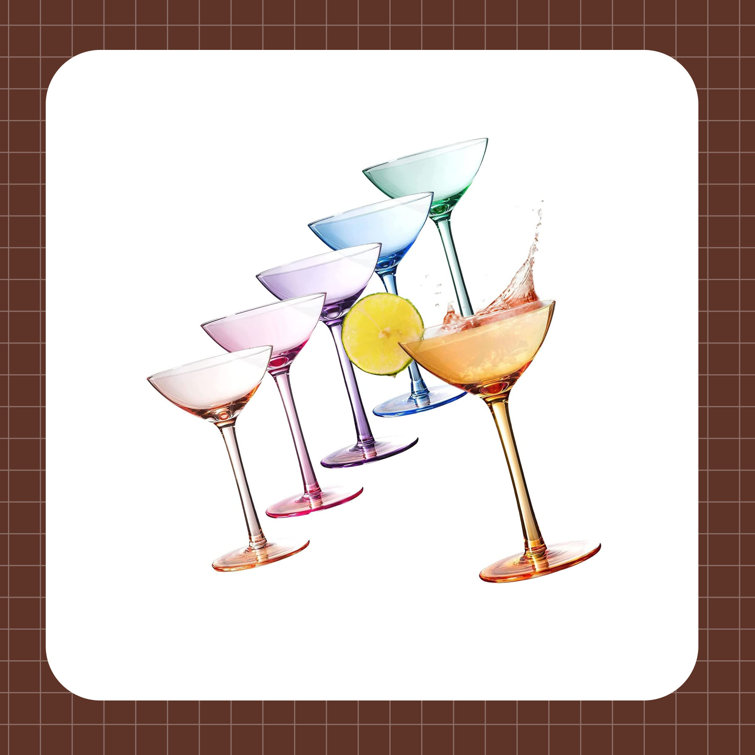The image features a square artwork with rounded edges, presenting a sequence of six cocktail glasses, each tilted and sitting atop a white background adorned with a brown grid pattern. From back to front, the glasses are tinted in diverse hues: green, blue, purple, pink, and light red. The largest glass, positioned to the side, contains an orange liquid and is garnished with a lemon wedge on its rim. The glasses exhibit a splash of liquid, adding a dynamic touch to the composition.